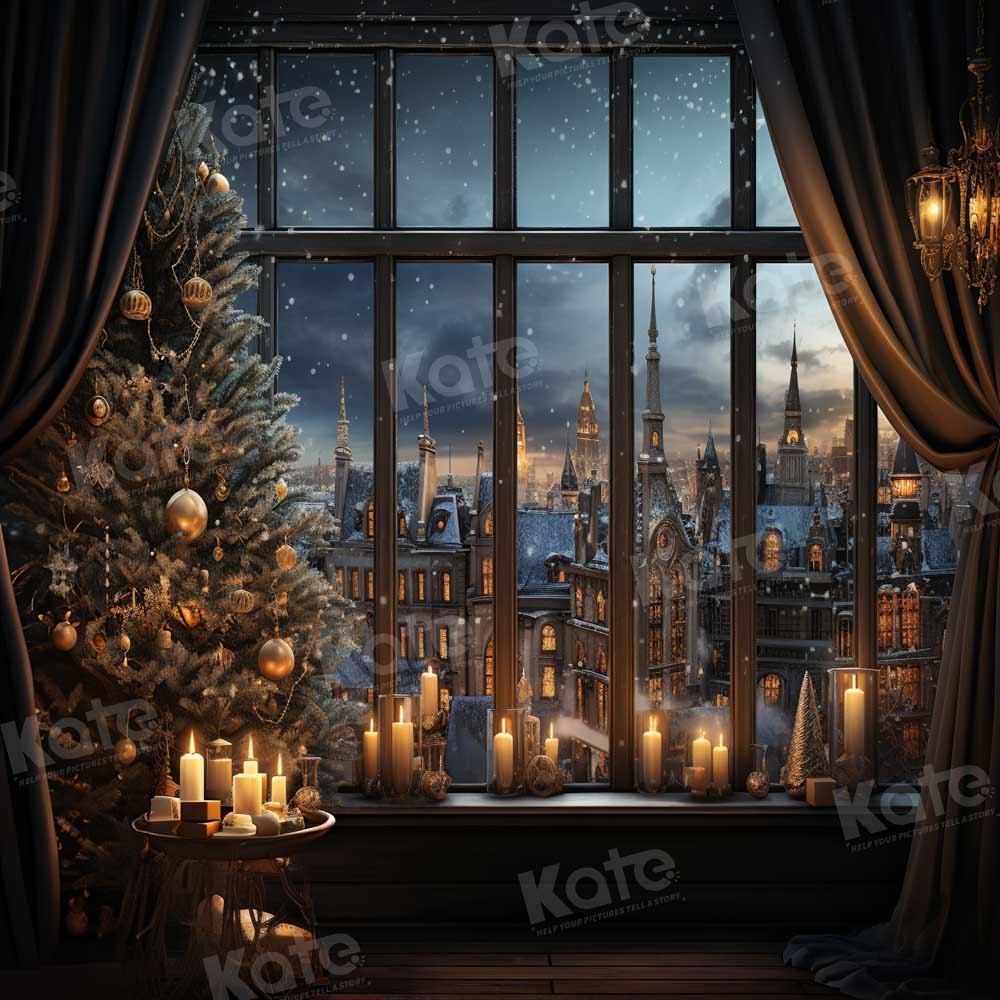This detailed drawing or painting captures a Victorian or Edwardian-era cityscape at night as viewed from a warmly lit interior. The room features reddish-brown curtains framing a large window divided into six long, rectangular panes. To the left of the window stands a richly decorated Christmas tree adorned with gold and silver ornaments and tinsel. Nearby, a small table brimming with lit candles adds to the cozy ambiance. The wooden windowsill itself holds an array of about a dozen lit candles, their warm glow blending with the light from a golden lamp with two bulbs hanging from the ceiling.

Outside the window, the cityscape reveals an old European, likely English or London, setting characterized by numerous spires and a clock tower, bathed in various shades of gray and blue. The sky is dark, peppered with stars and softly falling snowflakes. Buildings in the distance illuminate the night, creating a Dickensian Christmas atmosphere. The image is subtly watermarked with the name "Kate" in multiple locations.